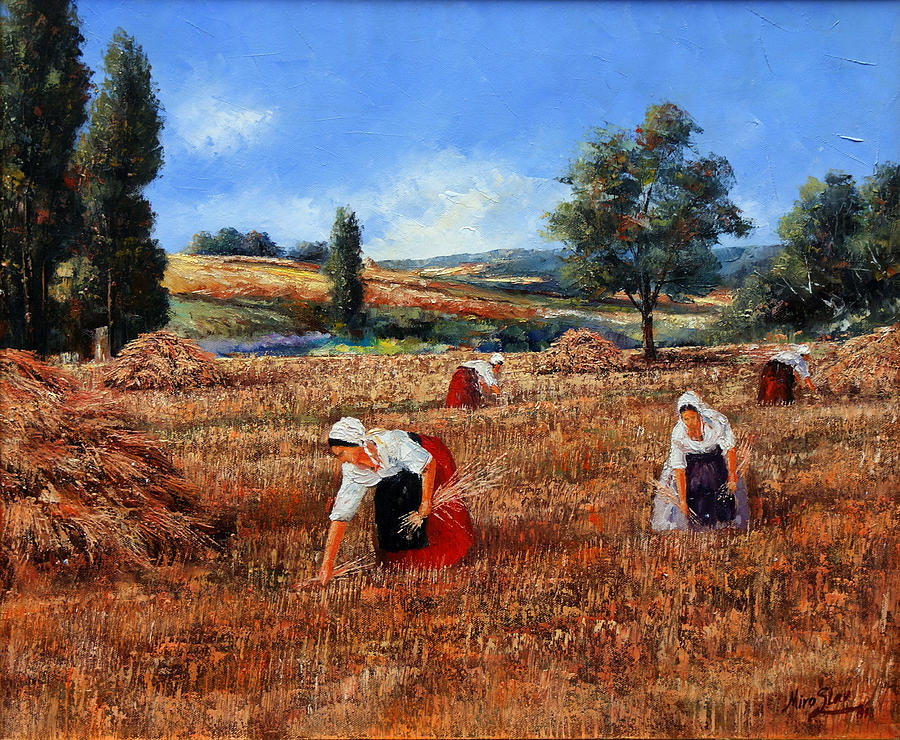This painting depicts four women, dressed in older-style clothing that suggests an Amish resemblance, working in a vast wheat field under a bright blue sky with minimal clouds. All women are wearing white shirts and white bonnet-like garments covering their heads. Three of them are clad in long red skirts with black aprons, while the fourth woman is distinguished by her light blue skirt and dark purple apron. The wheat field, the primary focus of the painting, occupies most of the foreground. In the background, rolling hills stretch across the horizon, framed by tall trees, smaller bushes, and reddish-brown foliage that accents the scenery. The sky, clear and blue, enhances the sense of a sunny day, punctuated by a few wispy white clouds.